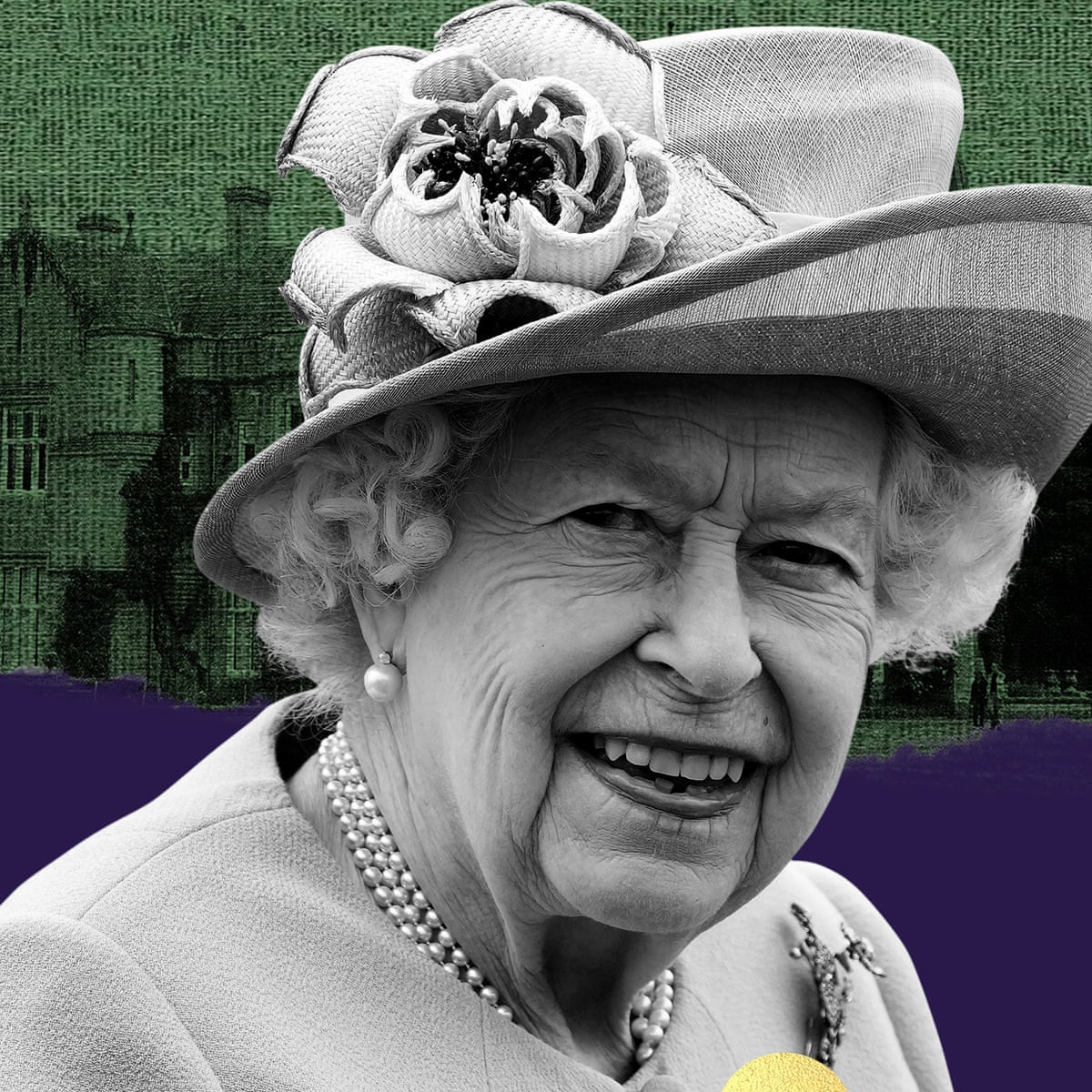This black and white photograph captures a dignified portrait of the late Queen Elizabeth, showcasing her from the upper chest up. She radiates elegance with a graceful smile that reveals her upper teeth, subtly highlighting the wisdom carried in her age-wrinkled face. The Queen is adorned in a fancy hat embellished with a meticulously crafted fabric flower, likely a rose. Her short, white hair neatly frames her face and gently covers her ears, one of which is adorned with a delicate pearl earring. Complementing this, she wears multiple strands of pearl necklaces around her neck, adding to her royal poise. The background of the image exhibits a unique, computer-altered skyline of buildings in rich green tones, resembling green fabric, juxtaposed with a blue section below, adding a surreal yet sophisticated touch to the composition.